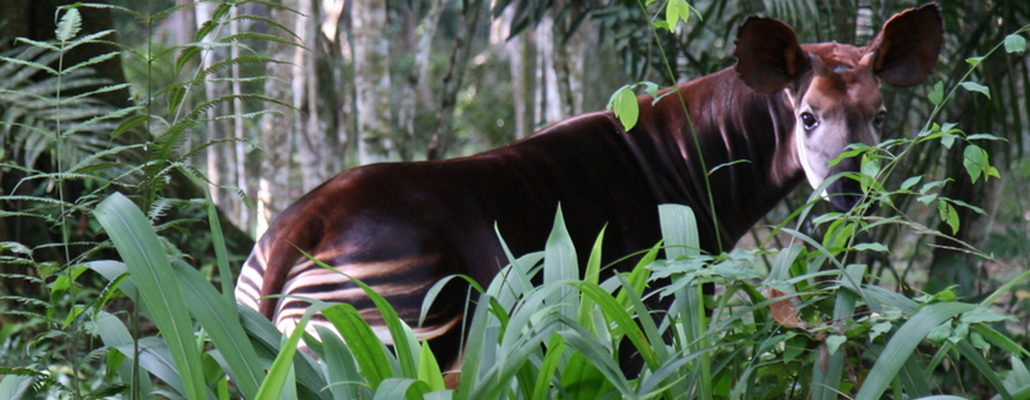In a dense forest setting, this long horizontal photograph captures a young deer-like animal, possibly a caribou, positioned with its body facing right and its head turned to engage directly with the camera. The animal's soft, shiny brown coat features distinct white markings on its face, with large, expressive round ears and a prominent black nose. The foreground is lush with ferns, grass, and twigs, while the background reveals a thick assembly of tree trunks. It stands near a giant rock, seemingly startled during its leaf-feeding amidst the greenery, ferns, and tall plants. The photograph is 4-5 times wider than it is high, emphasizing the forest's depth and the rich tapestry of vegetation surrounding the animal.